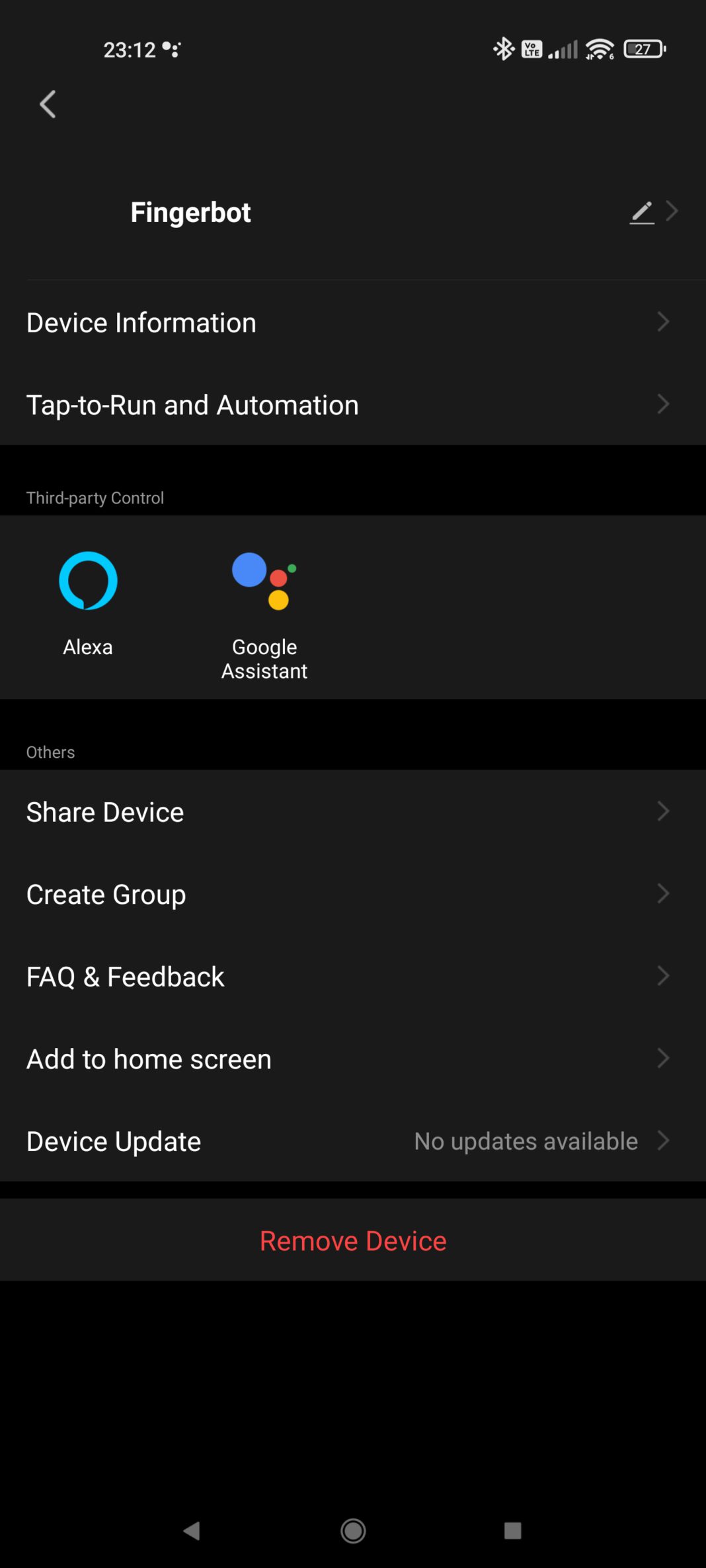A mobile phone screenshot displays various informational elements in a detailed manner. At the very top of the screen, there is a status bar presenting device details in white font: the time is 23:12, the Bluetooth icon is present, and the mobile signal strength shows two out of six bars. Additionally, full Wi-Fi connectivity is indicated, alongside a battery icon displaying 27% remaining battery. 

The screenshot is in dark mode, providing a black background with white text overlay. An open menu titled "Fingerbot" is visible, followed by sections labeled "Device Information," "Tap-to-Run and Automation," and "Third-Party Control." 

Within the "Third-Party Control" section, there's a lighter black rectangle containing icons for Alexa and Google Assistant. The Alexa icon is recognizable by its blue circle with a black chat bubble in the middle, while the Google Assistant icon consists of three differently colored circles.

Further down, another section labeled "Others" appears, listing options in white font including "Share Device," "Create Group," "FAQ and Feedback," and "Add to Home Screen."